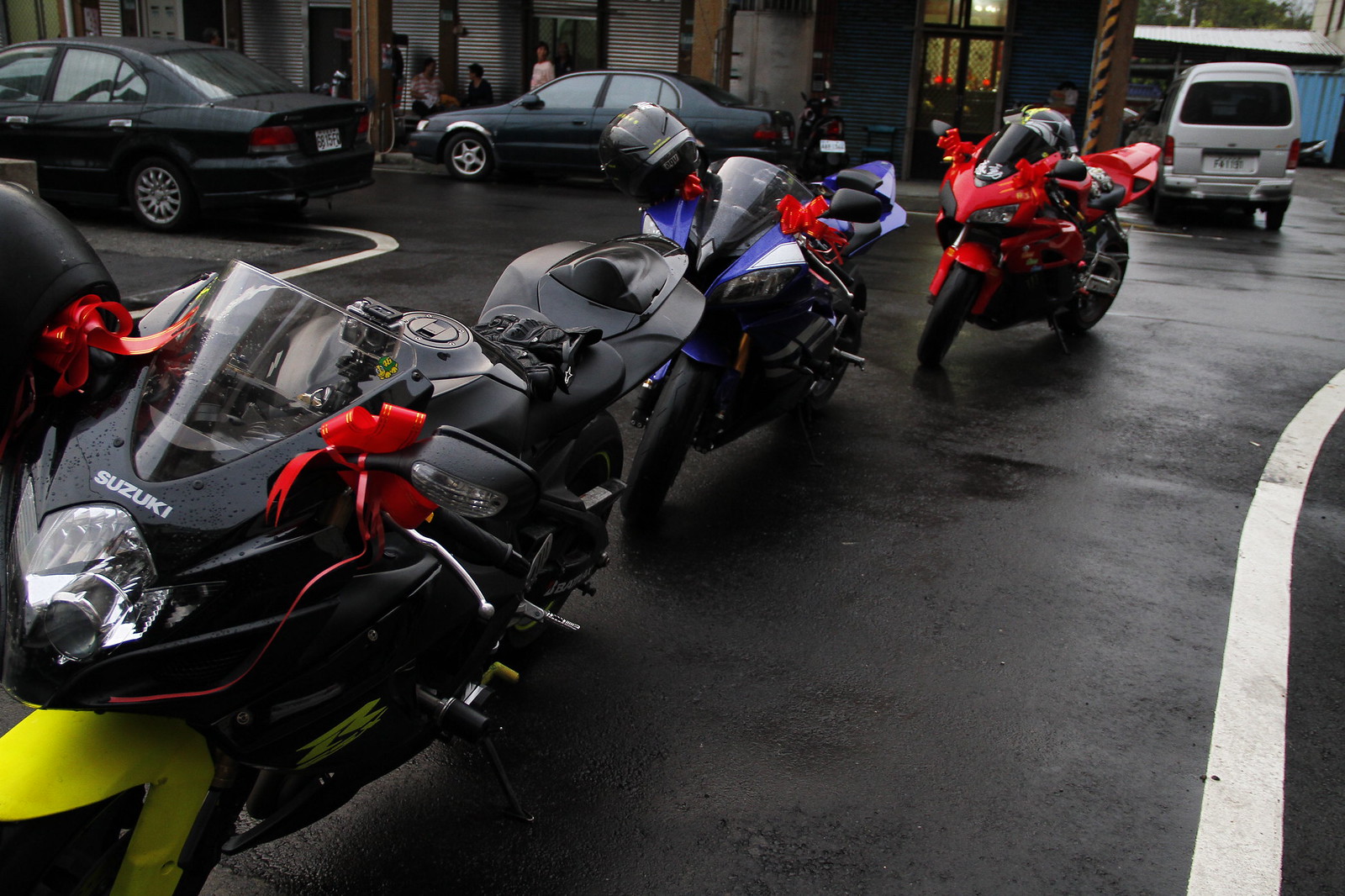This image captures a lineup of three motorcycles, perfectly aligned on what seems to be a rainy day on a busy street. The motorcycles are positioned on pavement, facing the camera. The foremost motorcycle is a striking black and yellow Suzuki, adorned with two red bows on its handlebars and a yellow wheel cover. Just behind it, another Suzuki sports a sleek blue and black color scheme, also featuring two ribbons on its handlebars, with a helmet dangling from the left handlebar. The final motorcycle in the lineup is predominantly black with vibrant red detailing and matching red bows on its handlebars. The motorcycles are neatly arranged in ascending order from the lower left to the upper right of the frame. In the background, several cars are parked, including a black car, a green car, and a white van. A few buildings and some pedestrians are visible, adding to the bustling ambiance of the street. A distinct white line runs up the right-hand side of the image, further emphasizing the scene's orderly nature.